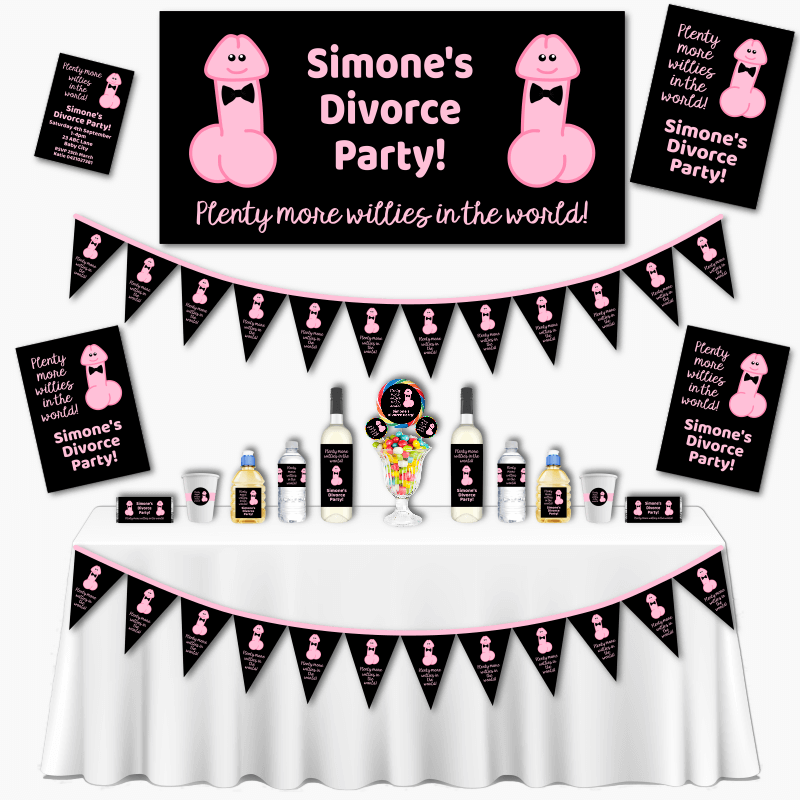This digital art image depicts a lively party scene celebrating Simone’s divorce. The lower half of the image features a rectangular table draped with a white tablecloth, adorned with small black triangular flag designs that echo the festive theme. On the table, a variety of items are meticulously arranged, including several glass bottles, cups, and a jar filled with colorful candies, alongside water bottles and liquor bottles.

Dominating the upper section of the image is a series of posters and banners that vividly communicate the party's theme. The central horizontal black poster, adorned with pink text, reads “Simone’s Divorce Party” in bold letters, flanked by playful icons resembling pink men’s private parts, each donning a black bow tie, black eyes, and a darker pink mouth. Beneath the main message, an additional line reads, “Plenty More Willies in the World.” Similar posters are aligned vertically on either side of the main poster and continue down the wall, reinforcing the celebratory theme. The repeated pink-on-black text and whimsical icons create a cohesive and festive atmosphere throughout the image.